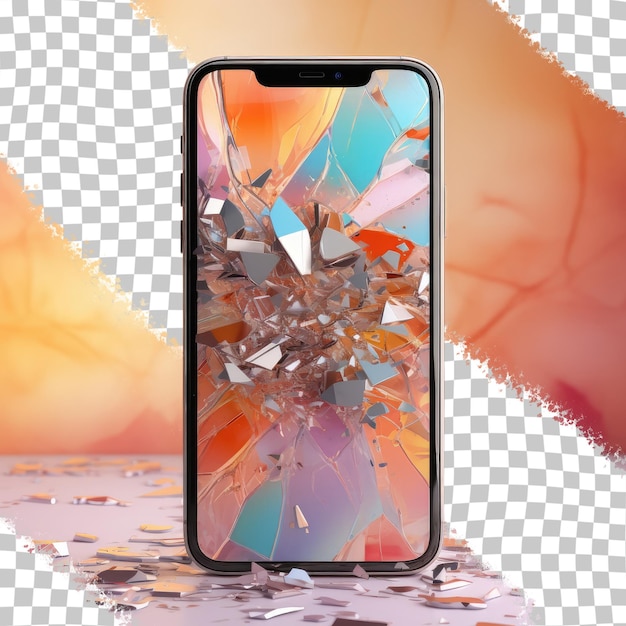The image depicts a vertically positioned phone at the center, with its front screen shattered, leaning against a vibrant backdrop. The phone is surrounded by numerous shards of glass, both on its surface and scattered around the floor or table it rests on. The screen displays a mix of pastel colors such as oranges, purples, light blues, and greens. This artistic composition features a background primarily in shades of yellow, orange, and red, transitioning to more yellow hues towards the upper left. There are three diagonally positioned checkered stripes in light gray and white—one prominent stripe running from the upper left to the lower right, and smaller visible sections in the upper right and lower left corners. The entire scene has an art-piece quality, with the backdrop adding layers of depth and color, accentuated by shards of glass reflecting light. The surface beneath the phone appears to be a light lavender shade, further contributing to the colorful and intricate nature of the image.